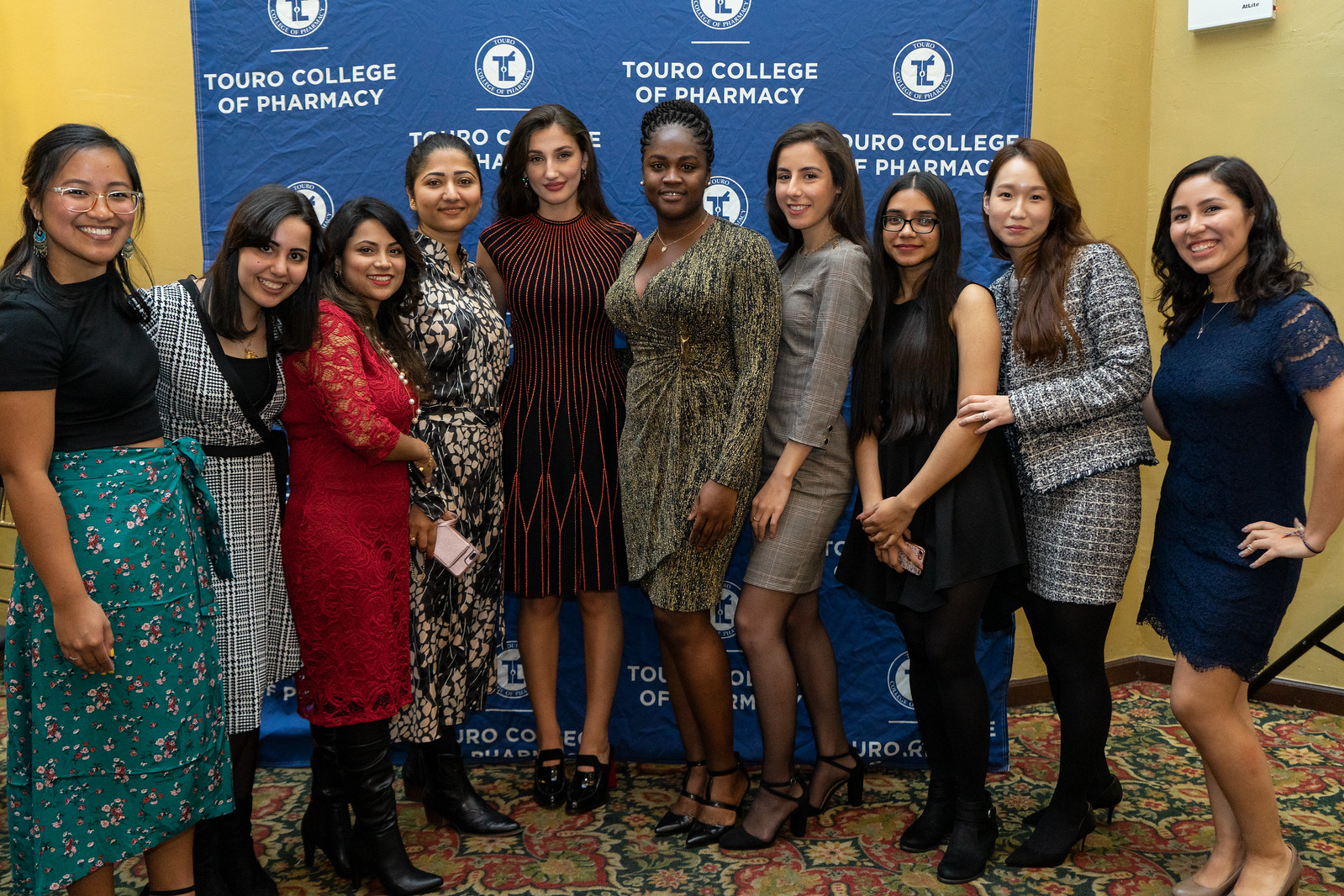This image depicts a group of ten women standing side-by-side, posing for a formal photograph within a yellow-walled room at Touro College of Pharmacy. The women represent a diverse array of ethnicities, including Hispanic, African-American, white, Asian, and possibly Indian. They are all dressed in elegant attire, featuring dresses, skirts, heels, and boots, suggesting a special occasion like a graduation party or a reunion. Behind them hangs a striking blue tapestry, bearing the college's name, "Touro College of Pharmacy," in white text, along with the college logo featuring the letters "TC." The floor beneath them is covered with a richly patterned red carpet adorned with intricate floral designs, reminiscent of a hotel setting. Overall, this vibrant and detailed photograph captures a moment of celebration and unity among the women at the college.